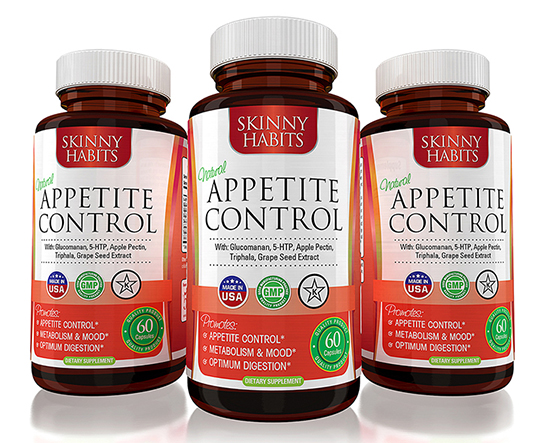This meticulously composed photograph showcases three identical jars, strategically arranged against a pristine white background with a reflective surface beneath. The polished setting suggests that this image is intended for an online marketplace. Each jar, crafted from brown plastic, is topped with a white screw-off lid. Positioned slightly ahead of the others, the central jar subtly stands out. The jars feature a distinctive white label, accented with a red square at the top, which bears the brand name "Skinny Habits" in bold white lettering. Directly below, in a smaller black font on a white square, the label reads "Appetite Control." Additionally, the labels include concise information in fine print, accompanied by three icons denoting "Made in the USA," "Genetically Modified Free," and another emblem that emphasizes the product's attributes. The image encapsulates a professional presentation, ideal for enticing potential buyers.